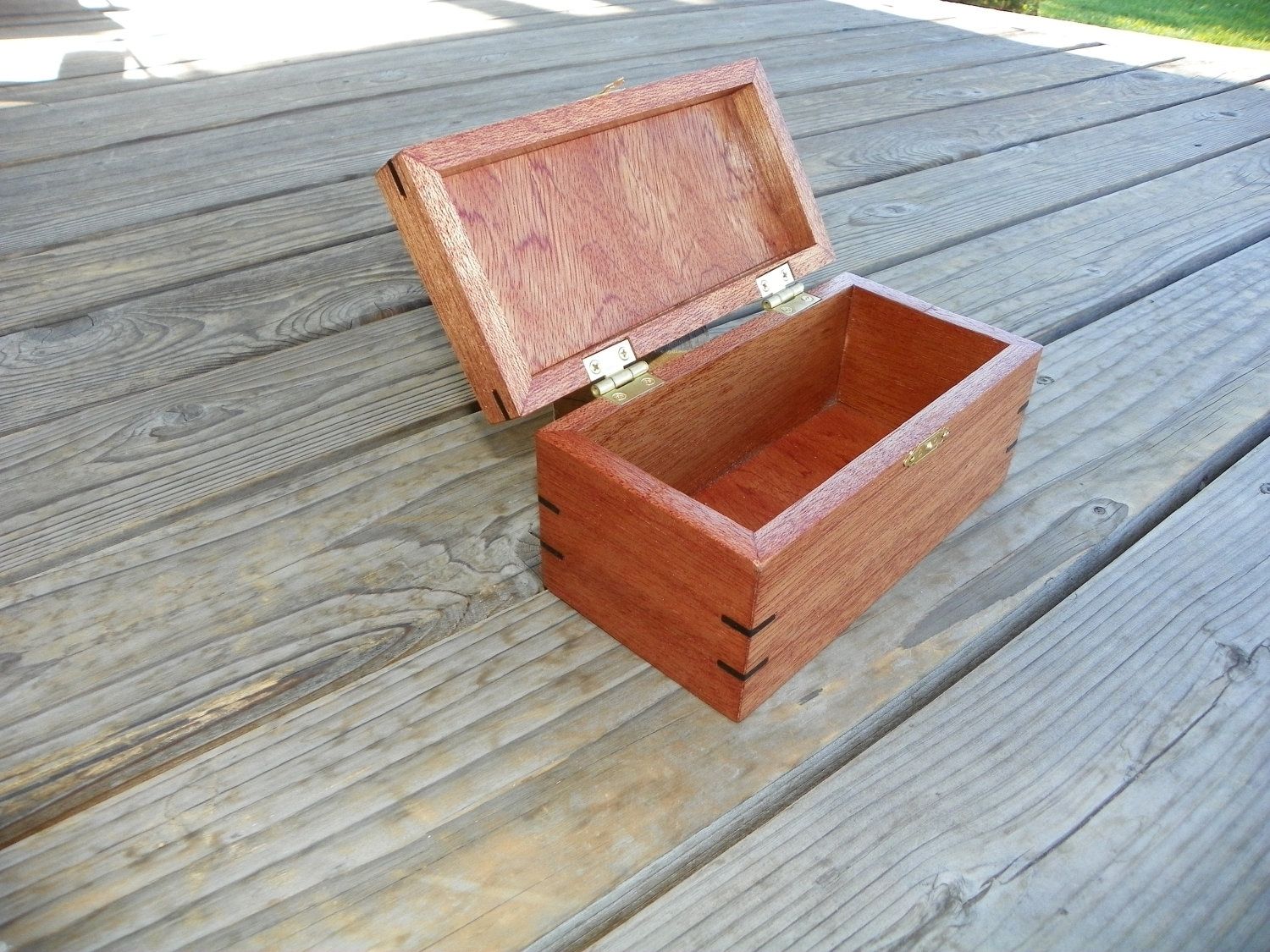This photograph, slightly wider than it is tall, captures a small, open wooden box resting on what appears to be a picnic table or wooden patio. The weathered wood of the patio is a light grayish color with long planks oriented from the lower left to the upper right of the image. The grains in the wood run in the same direction. The top left and top right corners of the patio are illuminated by sunlight, while the rest of the scene is in partial shade. In the top right corner, a small patch of grass is visible beyond the patio.

Centrally positioned, the rectangular, landscape-oriented wooden box is angled diagonally, with its left front corner facing the viewer. The box is made from a reddish wood and is approximately three to four inches tall, four to five inches deep, and about eight inches in length, though these dimensions are estimated. The lid is open, revealing a similarly colored wooden interior that appears to be empty. The lid is attached with gold, copper-colored hinges, adding a touch of contrast to the natural wood tones.